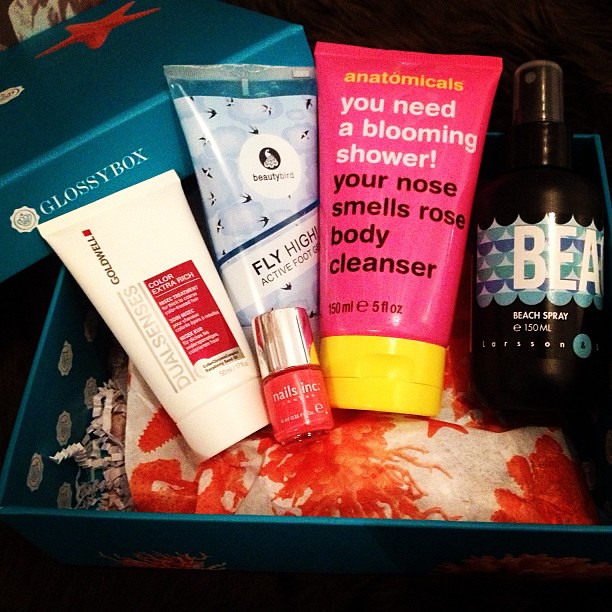This image features a detailed display of various beauty products arranged inside a turquoise-colored Glossy Box, a beauty subscription service container. The products include a mix of lotions, sprays, and nail polish, each in a distinctive bottle or tube. 

On the far left is a product from Goldwell Dual Senses, housed in a white bottle with red lettering. Next to it is a foot gel by Beauty Bird labeled "Fly High Active Foot Gel." In the center is a large pink tube with a yellow cap from Anatomicals, featuring the text "You Need a Blooming Shower" and "Your Nose Smells Rose Body Cleanser" in white and dark lettering respectively. To the right is a dark brown bottle of beach spray with blue and white text indicating "Beach Spray." Finally, there is a smaller nail polish bottle from Nails Inc in a pinkish-red hue.

The products are neatly arranged in the Glossy Box, with the box lid visible in the top left corner, showcasing its distinctive turquoise color. Also included in the packaging is orange and white gift wrapping, adding a festive touch to the display. The vibrant assortment of colors and variety of products suggests a curated selection ideal for beach outings or personal pampering.